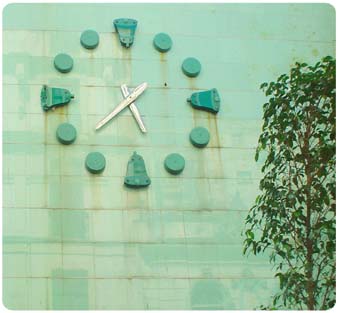This image captures a unique clock mounted on a brick wall. The clock is characterised by a series of dark green squares arranged in a circular pattern directly on the wall, blending seamlessly with the bricks. The hour and minute hands are clearly visible, providing the time for those who can read an analog clock. The design omits traditional clock face features such as numerals and a defined boundary, making it a minimalist and artistic interpretation of a timepiece. This clock's aesthetic might pose a challenge for young children to understand, as it lacks prominently distinct markers. The overall look is simple yet intriguing, showcasing a blend of function and form.